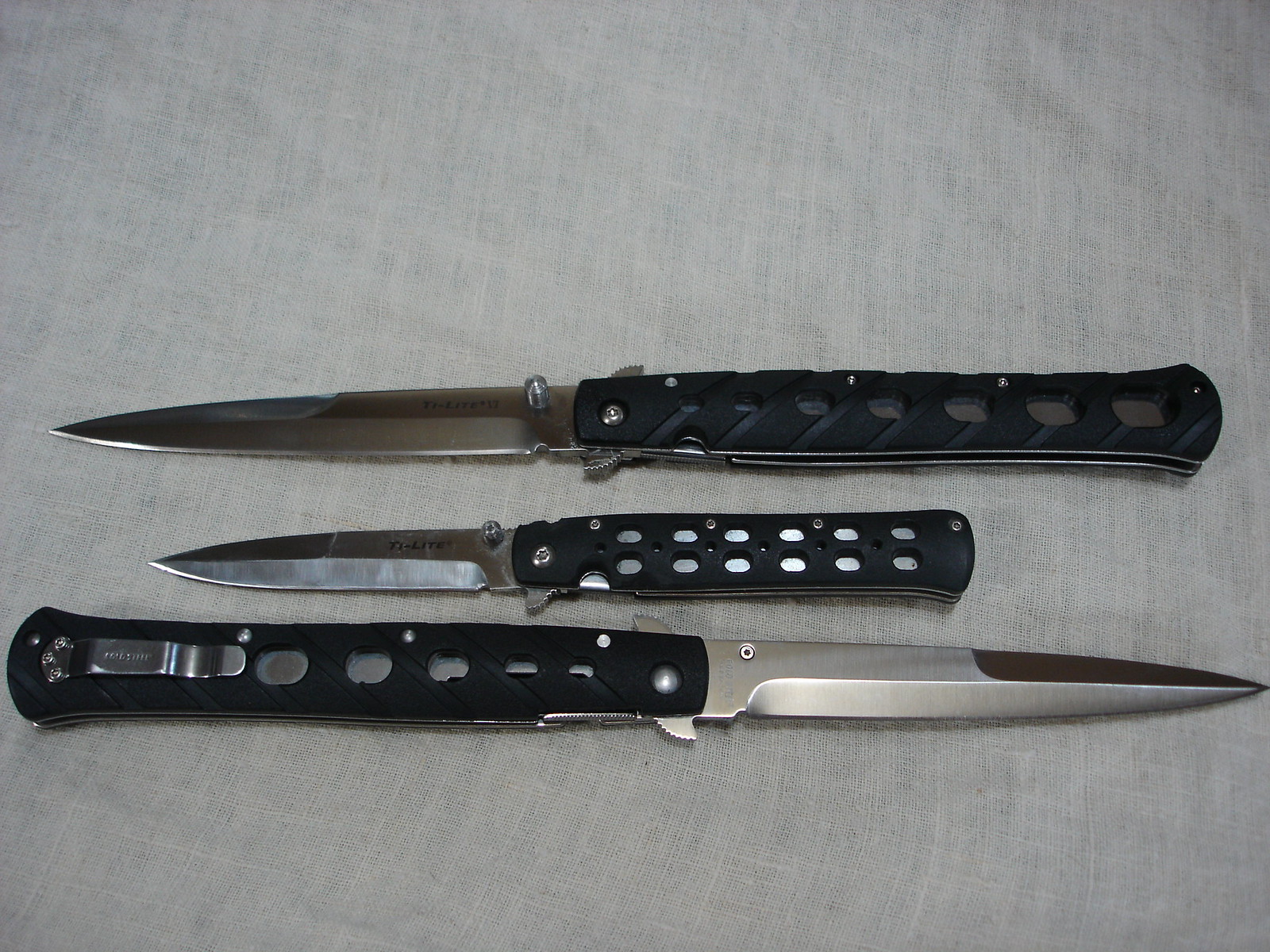This is an amateur photograph of three switchblade knives, positioned horizontally on a light gray sheet of linen. The knives are almost dead center in the frame, dominating about a third of the image. The top switchblade has its shiny stainless steel blade, approximately five inches long, extended to the left, while its black handle with cutouts, revealing the blade, rests to the right. The middle knife, the smallest at around three inches long, mirrors this orientation with its blade also sticking out to the left and its handle to the right. This knife has a similar black handle with visible cutouts. The bottom knife, the largest, extends almost fully from one edge of the image to the other, with its stainless steel blade, roughly six inches long, pointing to the right and its handle on the left. All three knives feature a beveled blade design and a two-sided mechanism for opening and closing. There are no marks, date stamps, or text, conveying a sense that these might be used items potentially listed for sale on a site like eBay. The overall sharpness and detail of the blades are evident in the imagery.